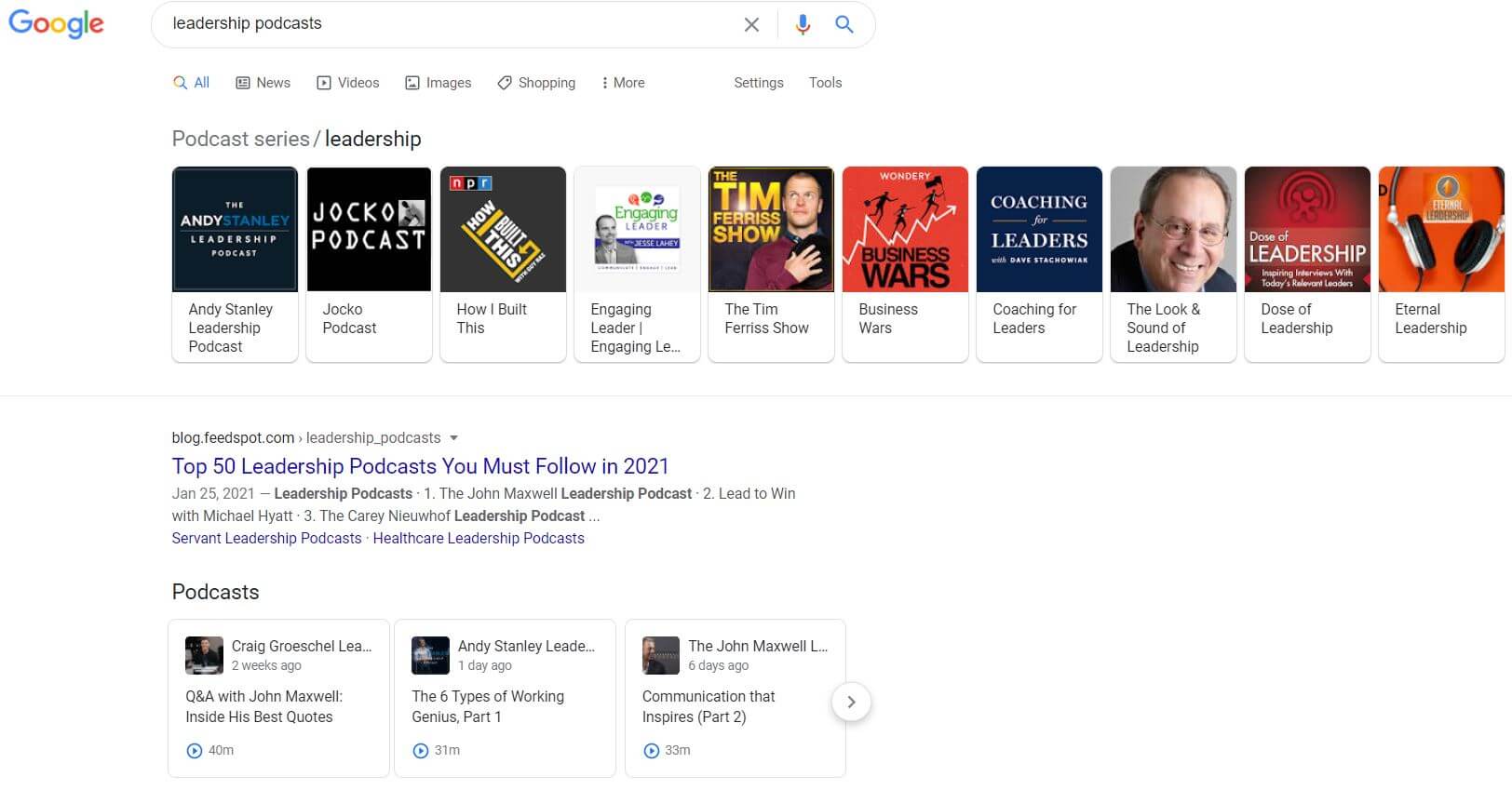The image displays a Google search engine results page characterized by a white background. At the top left, the iconic Google logo is prominently displayed with its distinct color scheme—blue G, red O, yellow O, blue lowercase g, green l, and red e. To the right of the logo is the search box, where the term "leadership podcasts" has been entered.

Beneath the search box, a menu bar spans from left to right with various options: "All," "News," "Videos," "Images," "Shopping," "More," followed by "Settings" and "Tools" towards the right. Below this menu, a section titled "Podcast series / Leadership" showcases a variety of podcast images. From left to right, notable podcasts include the "Andy Stanley Leadership Podcast," the "Jocko Podcast," "How I Built This," "Engaging Leaders," and "The Tim Ferriss Show," among others. Each podcast is represented by its unique and colorful image, some featuring photos of the hosts, such as Tim Ferriss on "The Tim Ferriss Show."

Further down, the first search result is from blog.feedspot.com, with the listing titled "Top 50 Leadership Podcasts You Must Follow in 2021."